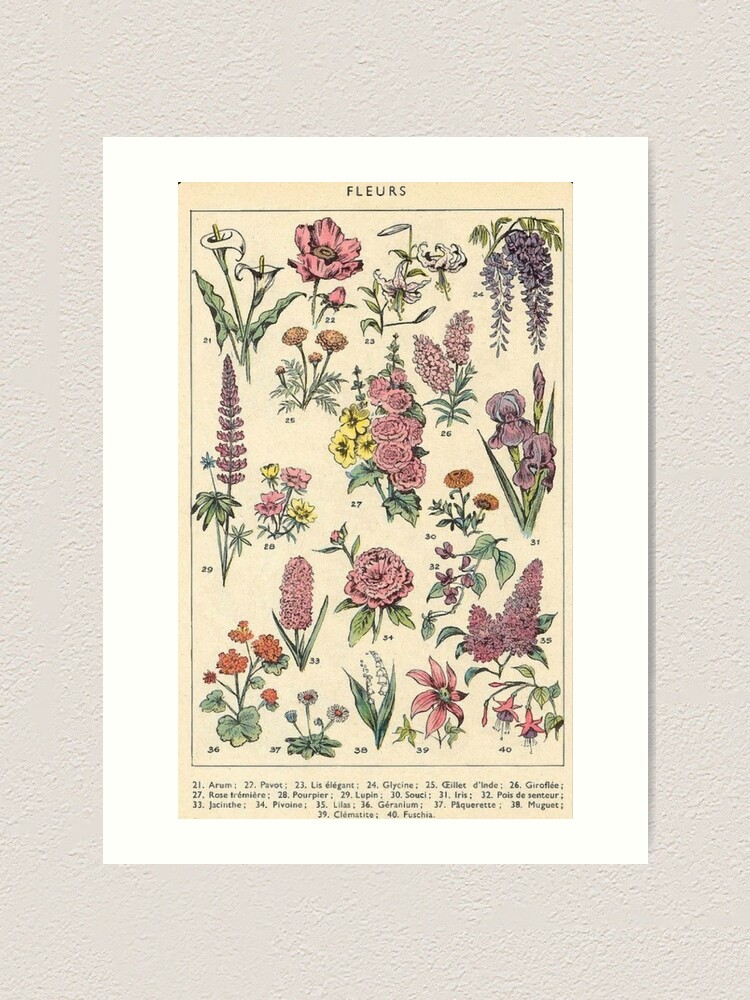A beautifully detailed scientific diagram is showcased in this photograph, which hangs on an ivory-colored wall within a white rectangular frame. The artwork, set against a faded orange-white sheet of paper, prominently features the word "FLEURS" at the top, spelled F-L-E-U-R-S. This striking illustration of flowers, ranging in numbers from 21 to 40, captures the diverse beauty of various plant species through intricate designs and vivid colors, including pink, yellow, blue, purple, and red hues. Each flower is meticulously labeled with its name and corresponding number, such as Aurum (21), Pathot (22), Lys Elgrond (23), Glycine (24), and continues through to Fuchsia (40). This classification system provides a glimpse into botanical variety, highlighted by the elegant French nomenclature beneath each illustration. The overall composition, set against a textured white drywall background, suggests a page extracted from an old botanical textbook, making it a captivating piece for admirers of floral artistry and scientific documentation alike.